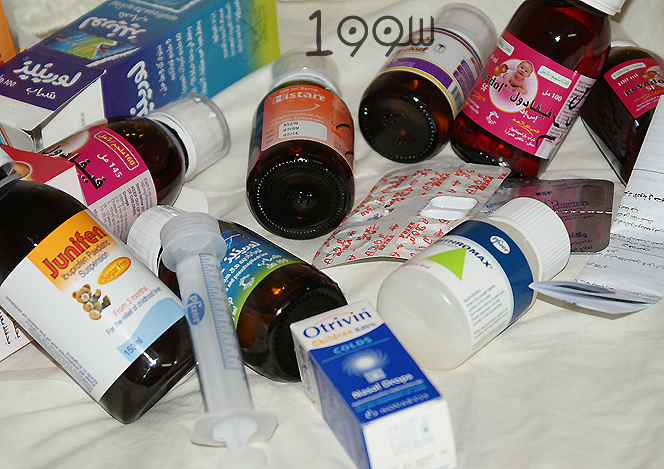This close-up photograph showcases a variety of baby medications scattered across a white bedspread. At the top center, the text "199W" is visible. There are eight bottles in total, most of which are made from dark brown glass, with one plastic bottle on the right side. The bottles feature labels in what appears to be Arabic script. Notably, one bottle labeled "JUNIFEN" with a teddy bear image indicates it is an ibuprofen pediatric suspension, sugar-free. Among the glass bottles, there are two red bottles with matching red labels and one red bottle with a purple label. Additional items include a blue box with white Arabic writing and a green bottom, another blue box reading "OTRIVIN Colds," some instructional paper pieces, and two blister packs — one centered and backed with aluminum foil, featuring red Arabic writing. Positioned above some of the bottles on the left side is a clear syringe marked with the word "Pfizer."